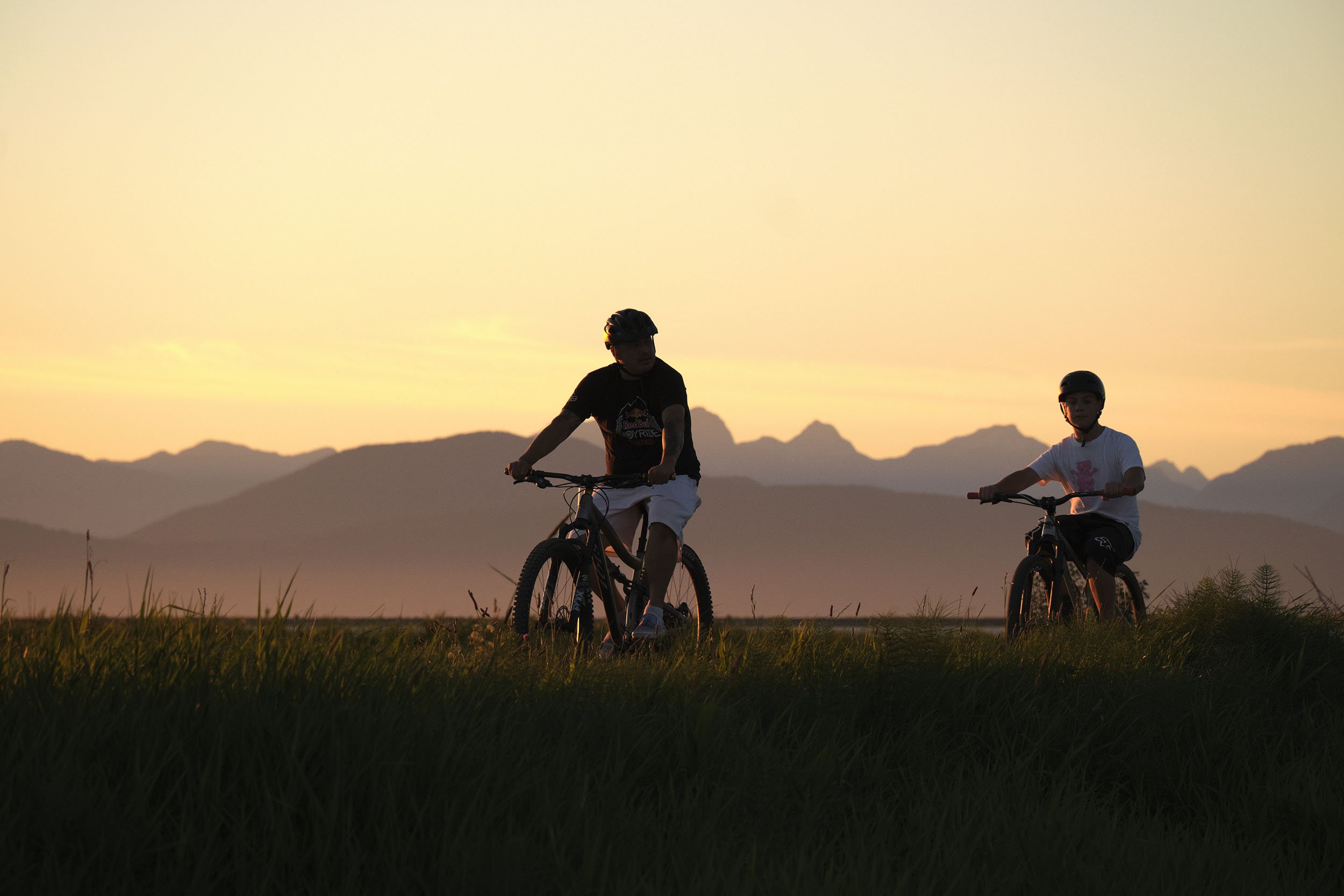The image features two cyclists riding along a barely visible path amidst lush, green vegetation. The scene is set against a stunning dusk backdrop, where the sky is an exquisite blend of yellows, peach, pink, and purple hues. Rising grey and purple mountains add depth to the background, while long grasses and dense foliage dominate the foreground. The leading figure appears to be an adult, possibly in his 40s or 50s, dressed in a black t-shirt with some indistinguishable writing, paired with light-colored pants, light sneakers, and a dark helmet. Behind him is a younger individual, likely a teenager or in his early 20s, sporting a white t-shirt with red text, black shorts, and a black helmet. The overall setting suggests a serene, yet slightly mysterious atmosphere, possibly owing to the onset of evening and a touch of fog enshrouding the mountains.